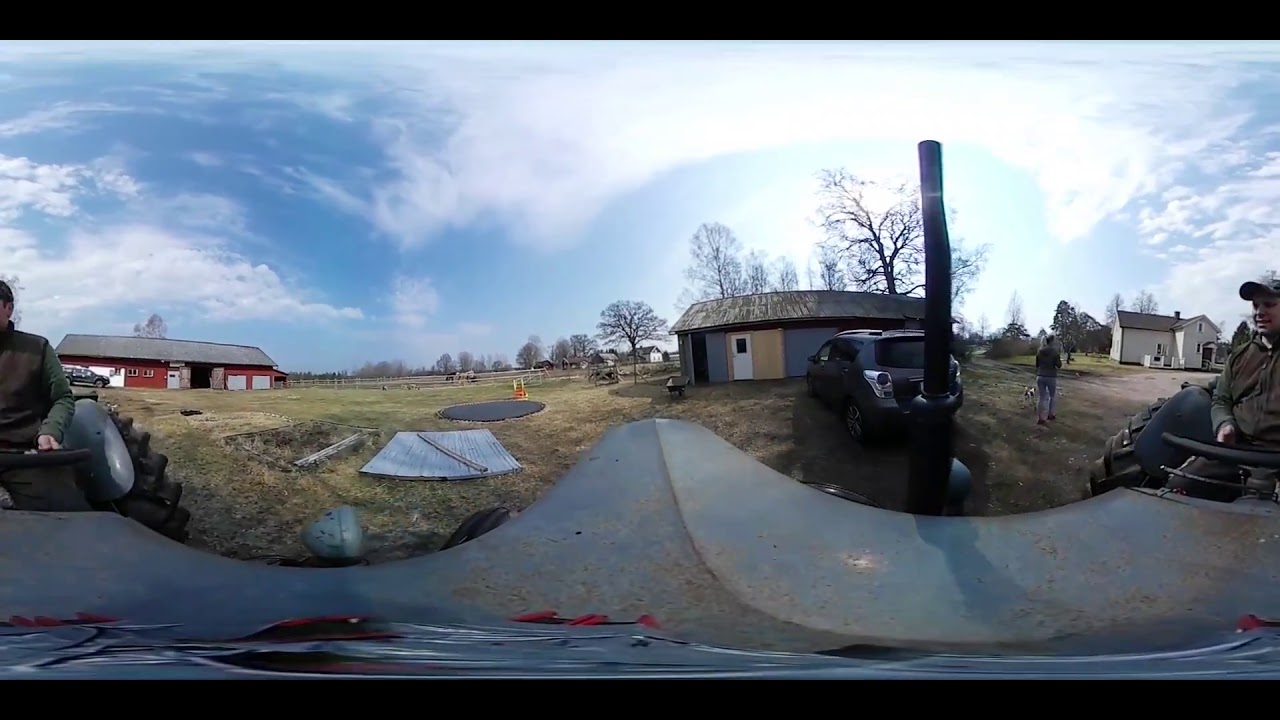In this panoramic, 360-degree image of a rural farm setting, various one-story houses and a two-story white farmhouse are depicted, surrounded by lush grass, trees, and open farmland. The sky, filled with some clouds, enhances the daytime atmosphere. In the center foreground, a gray tractor features prominently, with a man wearing a dark vest, green sleeves, and a light baseball cap, sitting at the wheel. Due to the panoramic effect, the same man appears on both the left and right sides of the image. To the left, there is a red barn with open doors, possibly indicating farming activities. Beside the barn is a small shed, and further left are horses in an open pen. On the right side, near a gravel driveway, stands the farmhouse, and a dark gray SUV or minivan can be seen parked nearby. A person with a small dog is also visible. Scattered materials, possibly for construction, lie in the forefront, suggesting ongoing or upcoming building work. The scene is vibrant with community life, with several people visible, appearing to prepare for farming or building activities.